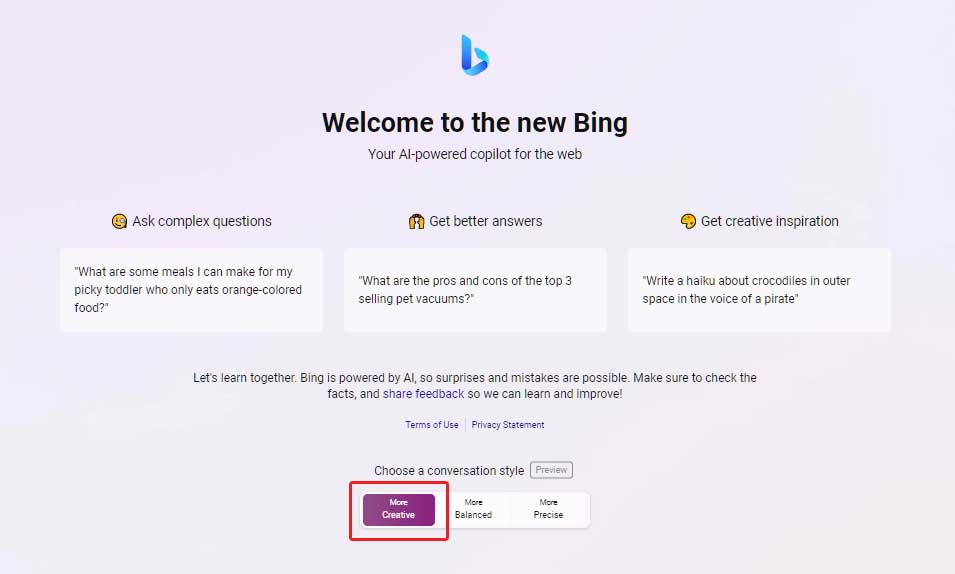The image features a large light purple background. At the top center, a small blue ribbon curls gracefully, displaying the text "Welcome to the new Bing, your AI-powered copilot for the web" in black print. Below that, in yellow, it encourages users to "Ask complete questions." 

A light-colored box further down reads, "What are some main meals I could make for my picky toddler who only eats orange-colored food?" In the center of the image, bold lettering states, "Get better answers," accompanied by illustrations of small yellow hands. It continues with an example query: "What are the pros and cons of the top three selling pet vacuums?"

Further down, the text invites creative thinking with "Get creative inspiration," again highlighted by a yellow hand illustration, accompanied by the prompt: "Write a haiku about crocodiles in outer space in the voice of a pirate."

The message "Let's learn together. Bing is powered by AI, so surprises and mistakes are possible. Make sure to check the facts," follows. In blue text, it encourages users to "Share feedback so we can learn and improve," with links to the "Terms of Use," a separator line, and the "Privacy Statement."

At the bottom, there’s a section inviting the user to "Choose a conversation style," with options in a purple box labeled "More Creative," highlighted in red, and other options reading "More Balanced" and "More Precise." The section also mentions "Preview" in a small box.